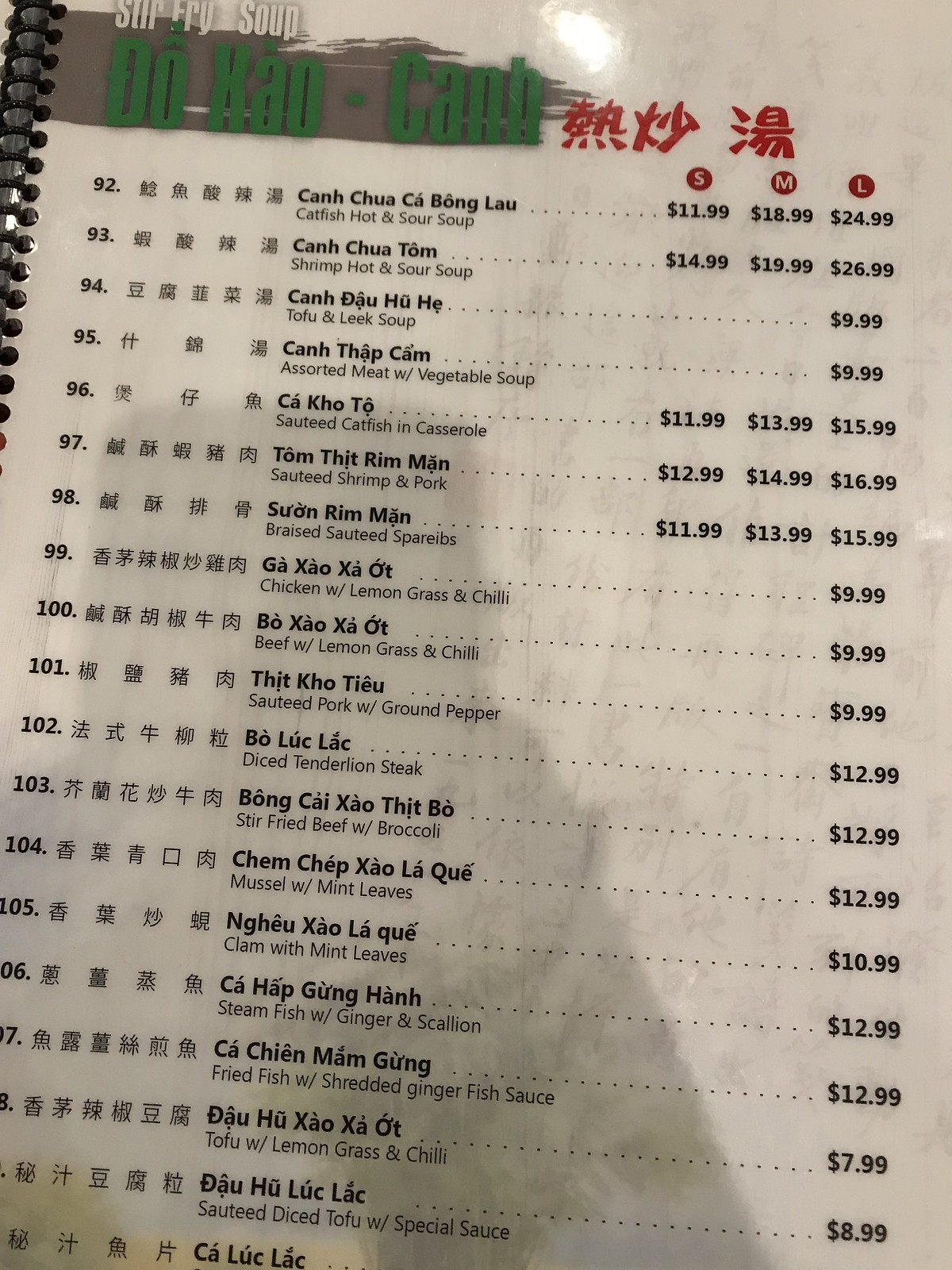A detailed photographic image of a white menu from an Asian restaurant. The menu features red characters at the top, with three prominent symbols. Below these characters, there is a gray banner displaying various categories, including "Do," "Cow," "Can," "Stir Fry," and "Soup." The menu is bound together by a metal strip.

The items listed on this page are numbered from 92 to 110, showcasing a variety of dishes available in different sizes: small, medium, and large. Notably, the first item on the list is "Kan Chua Ka Bang Lao" soup, which is a catfish hot and sour soup priced at $24.99 for a large serving. The most expensive item listed is "Kan Chow Tom," a shrimp hot and sour soup, priced at $26.99 for a large portion.

The menu also features some subtle shadows cast along its surface and includes faded drawings of characters, adding an elegant touch to its design.